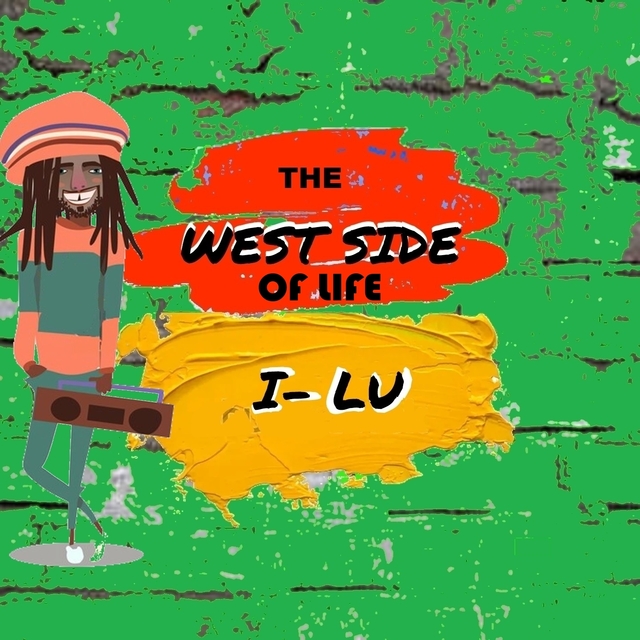The image appears to be a vibrant, urban-themed poster with a graffiti-like aesthetic. The background is a weathered, green-painted wall with visible cracks and hints of underlying wood, giving it a distressed appearance. In the center, there are two prominent paint splatters: a red one at the top and a yellow one below it, showcasing the textured, layered look of the paint. Inscribed within the red splatter are the words "The West Side of Life," while the yellow splatter contains the text "I-LB."

On the left side of the image is a cartoon-style figure that embodies a Rastafarian or Jamaican vibe. The character is a black female with long brown dreadlocks, wearing a large, orange-pink hat that covers her hair. She has a big, cheerful smile and is dressed in a sweater with aqua and pink stripes, paired with pants and some kind of footwear. Completing her hip-hop inspired look, she is holding an old-school boombox in one hand. The overall design and elements converge to create a lively, street-art-inspired scene.